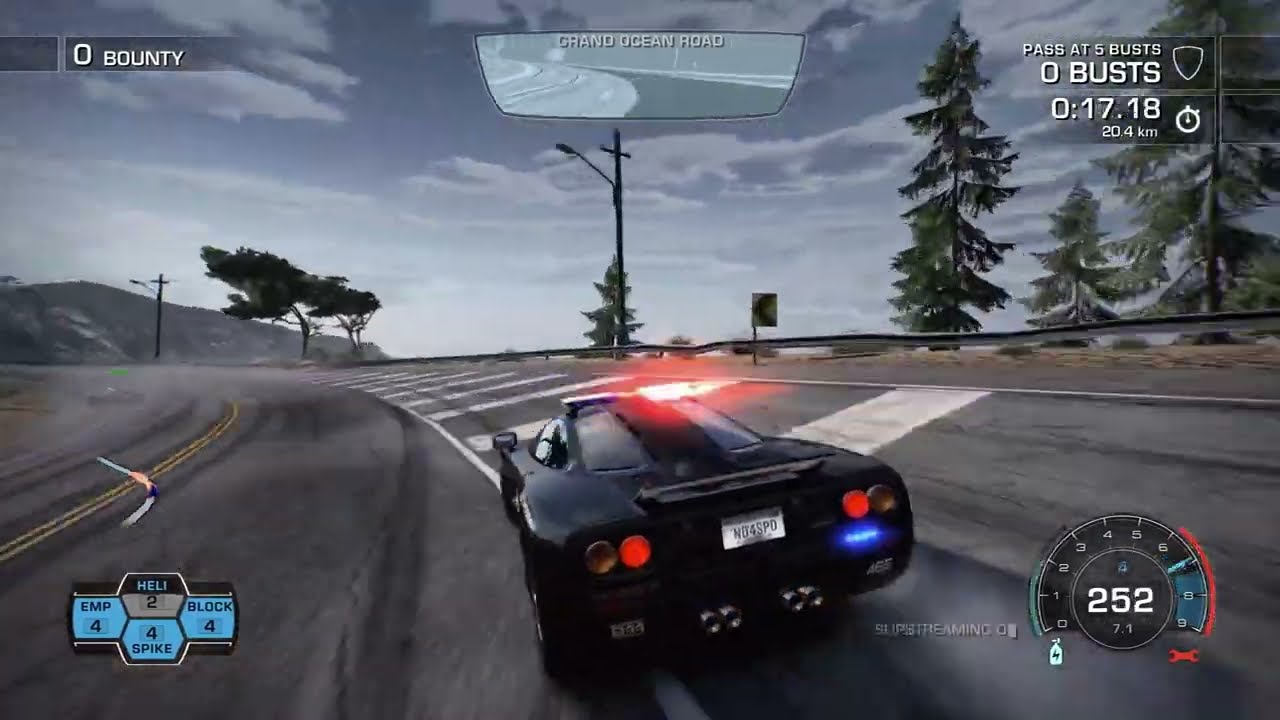The screenshot captures an intense moment from a racing video game, likely Need for Speed, showcasing a sleek black sports car barreling down a highway at 252 kilometers per hour. The car, viewed from behind, dominates the center of the image, displaying its rear license plate and illuminated brake lights as it makes a sharp left turn on a curvy road. The asphalt road features white stripes and a double solid yellow line, with guardrails on either side. Flanking the road are lush green trees, a hilly background, and an overcast cloudy sky. The car's speedometer, positioned in the lower right corner, confirms its high speed. In the top middle of the screen, a rearview mirror shows the text "Grand Ocean Road," while the top right corner displays relevant game information, including a timer showing 17 minutes and 18 seconds of driving time and a count of zero busts. Additionally, various game controls and characteristics are visible on the left-hand side of the screen.